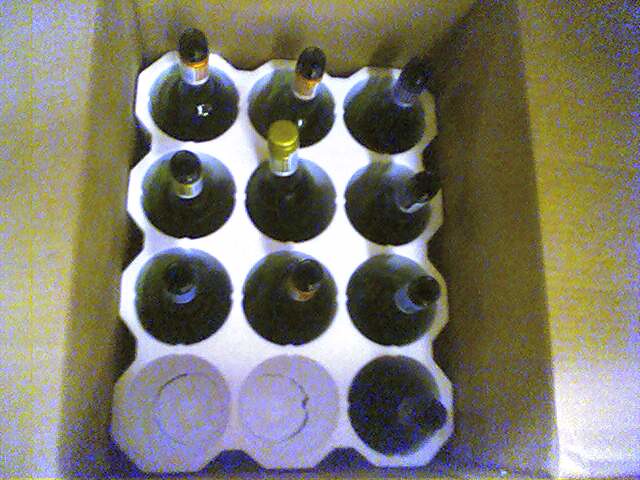The image is a poorly captured color photograph, exhibiting significant graininess, faded edges, and a soft focus, indicative of being taken with an old or low-quality smartphone camera. The viewpoint is from above, looking down into a cardboard box with partially visible flaps on either side. Inside the box, there's a white plastic or polystyrene holder designed to accommodate twelve wine or alcohol bottles. The holder has three horizontal rows and four vertical columns, with two bottles missing from the bottom left, leaving empty spaces. Only ten bottles remain, each topped with a variety of caps and labels: a mix of gold screw caps, different colored labels including blue, red, white, and orange—some bottles are capped, while others appear open. The box itself exhibits yellow splotches and noticeable fading, particularly pronounced on the right side, contributing to the overall blurriness and diminished image quality.